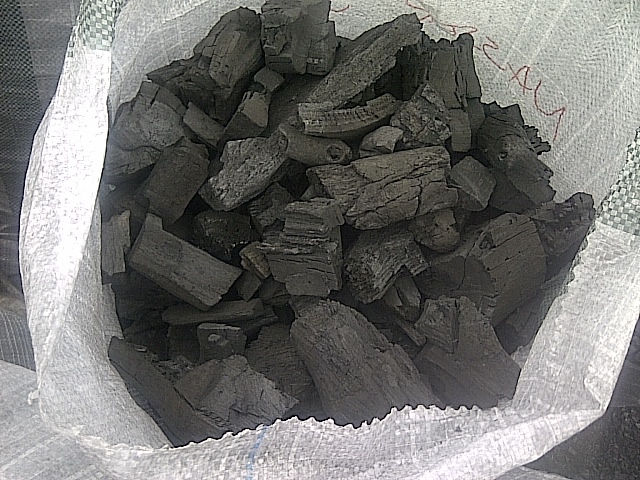The image depicts a netted, white plastic bag viewed from the top, containing 50 to 70 pieces of dark objects that resemble charcoal, burnt wood, or wood chippings. The objects vary in size from approximately two inches by four inches for the largest pieces to one inch by two inches for the smallest. The bag is about half full and shows a mixture of black and grey tones, suggesting the contents are primarily charcoal or similarly burnt material. The bag features an unclear label starting with 'UAS.' The image is predominantly in black and white, making it challenging to discern specific colors, but it appears that the bag is placed on a grey surface, possibly fabric, that might be a couch.